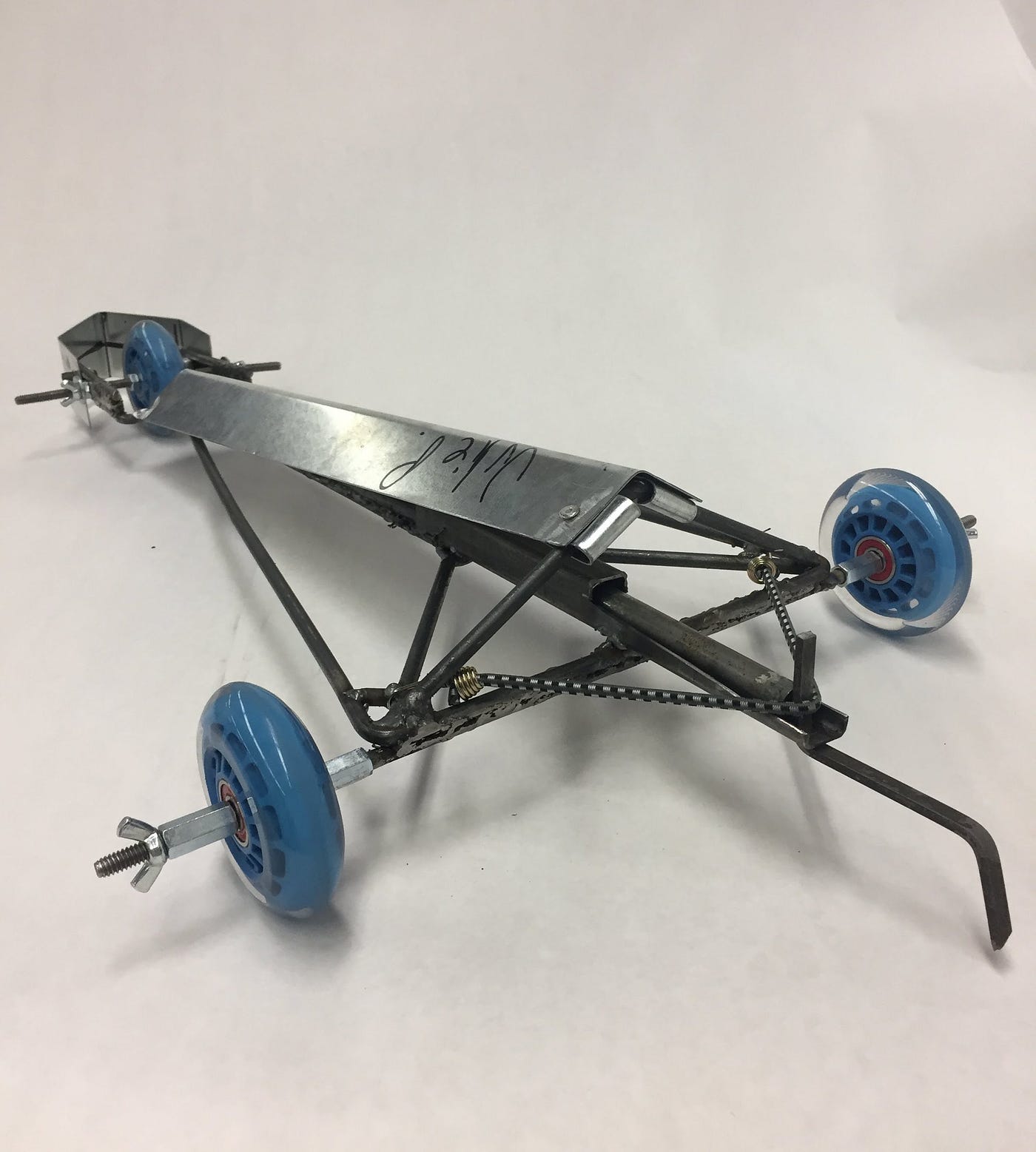In a stark white studio setting, the image showcases a unique homemade tricycle-like contraption. This interesting riding device features a black metallic frame and three blue plastic wheels reminiscent of skateboard wheels. The layout forms a large triangle, with two front wheels connected together and a single rear wheel, which is encased by a protective metal guard. The two front wheels are linked by an elastic string, presumably to aid in steering or stability, while a noticeable metal pipe extends and angles downward from the back. Silver nuts are visible holding the wheels in place, and there are a few black marker marks along the dark metal frame. Though the device lacks a seat, suggesting it might be designed for standing or requires an additional attachment, it overall gives a vibe of an intriguing and creative DIY project.